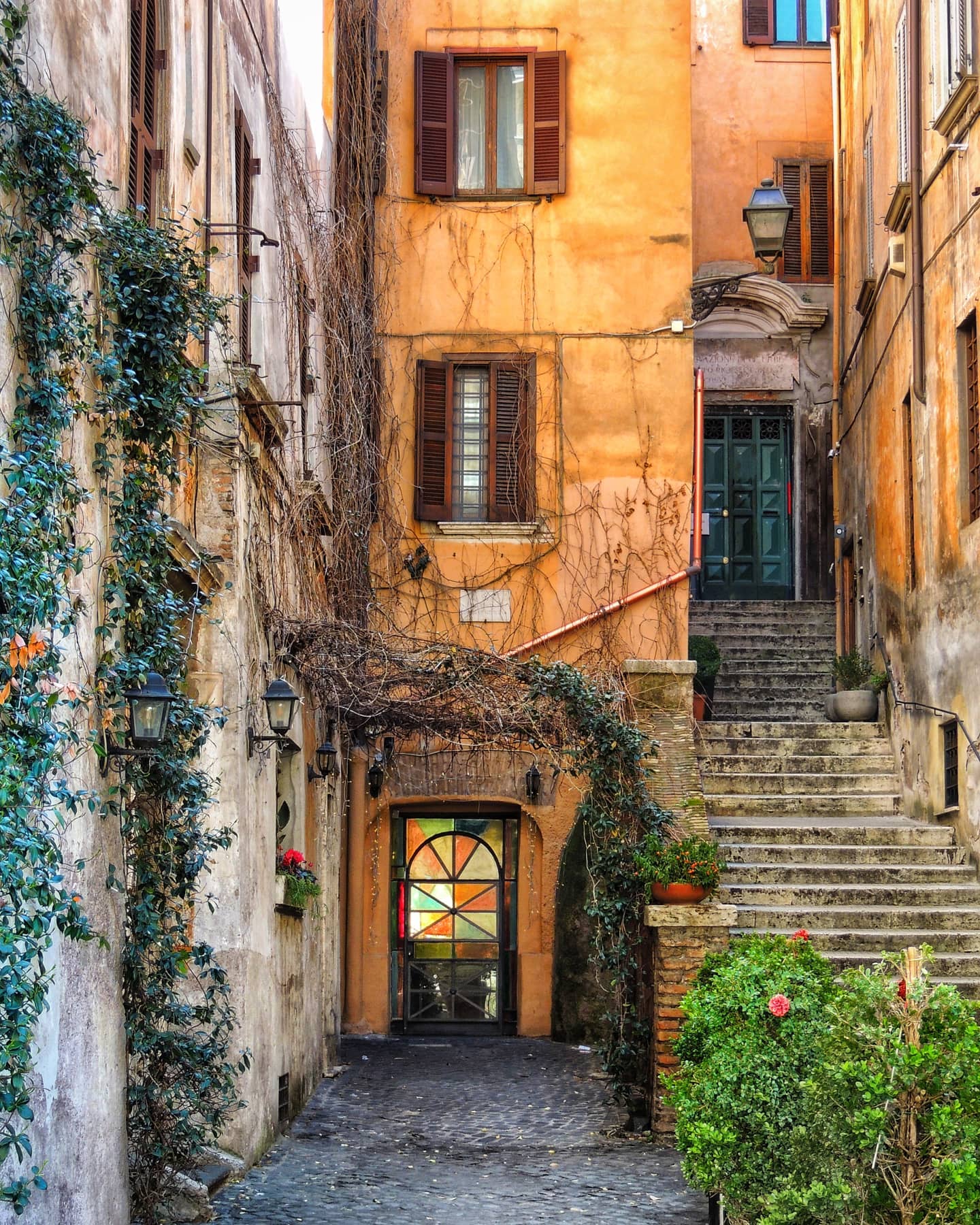The photograph is a professionally shot, full-color outdoor image taken during the daytime using natural light. It captures a vertically rectangular scene with a detailed view of a charming, older alleyway flanked by stone buildings. 

On the left side, there's a weathered stone building with a grayish hue, adorned with draping vines and flower pots on the window ledges. The center of the image features a brown stone building with an orange-toned wall. At ground level, a walkway leads to a brown door with a multicolored stained glass arch, further accentuated by vines that climb up the wall. Above this door, two sets of partially open windows can be seen on each floor.

On the right, there's a cement-plastered staircase leading up to a green door, adjacent to the brown building. Above this entrance, a street lamp adds a quaint touch. The bottom right corner of the image showcases a lush green shrub with vibrant pink flowers, while vines elegantly drape over the staircase and the buildings. The alleyway itself is dark gray, highlighting the aged yet picturesque character of the scene.